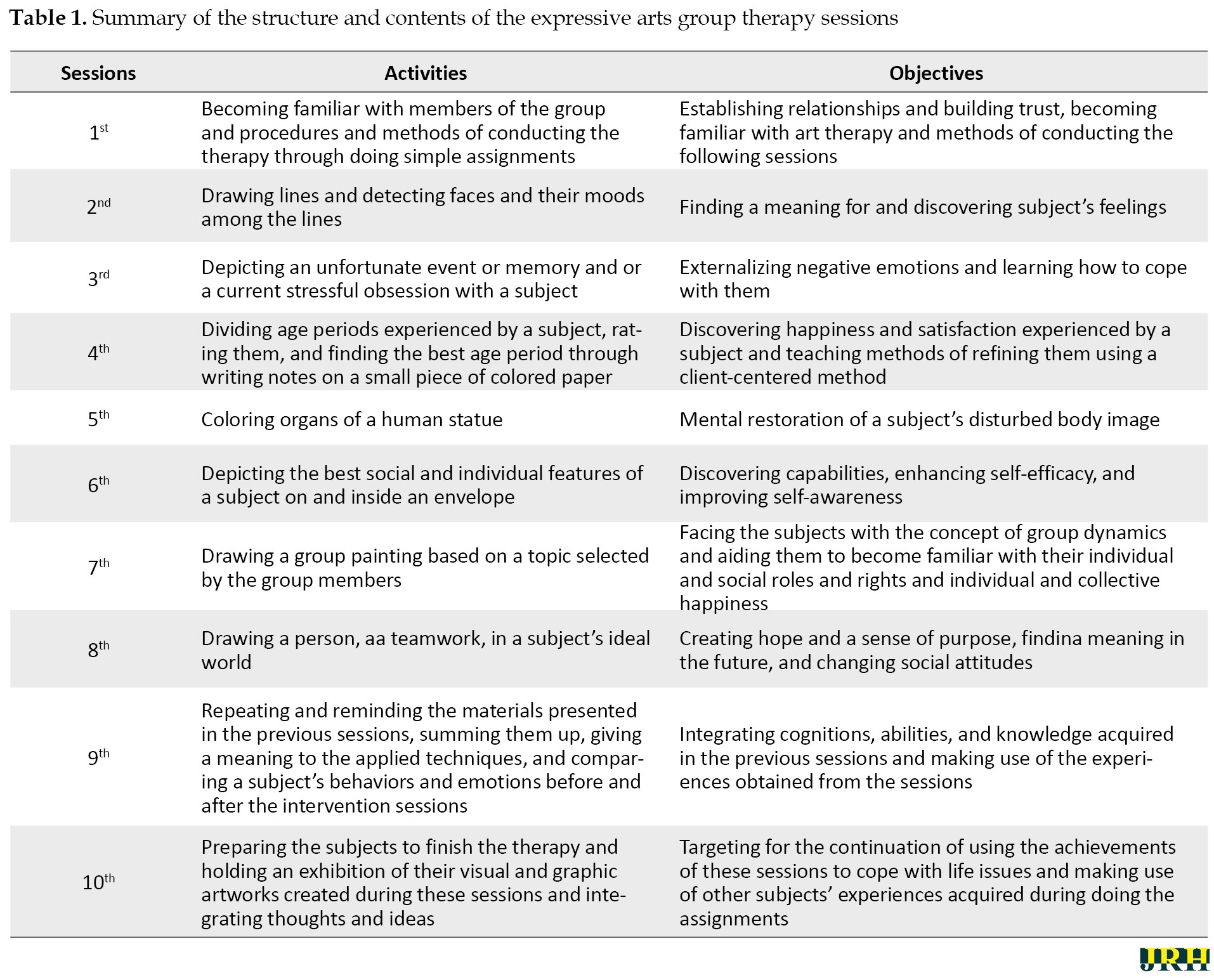The image is a black-and-white table titled "Table 1: Summary of the Structure and Contents of the Expressive Arts Group Therapy Sessions," appearing to be from a textbook or article. The table is rectangular, with the long sides as the horizontal edges, and features three columns labeled "Sessions," "Activities," and "Objectives" in bold black font. There are ten rows beneath these headers, each row alternating between white and gray with black text. The "Sessions" column lists sessions one through ten. The "Activities" column details specific expressive arts group therapy activities for each session, while the "Objectives" column outlines the goals associated with these activities. There is an additional logo in the bottom right corner labeled "JRH."